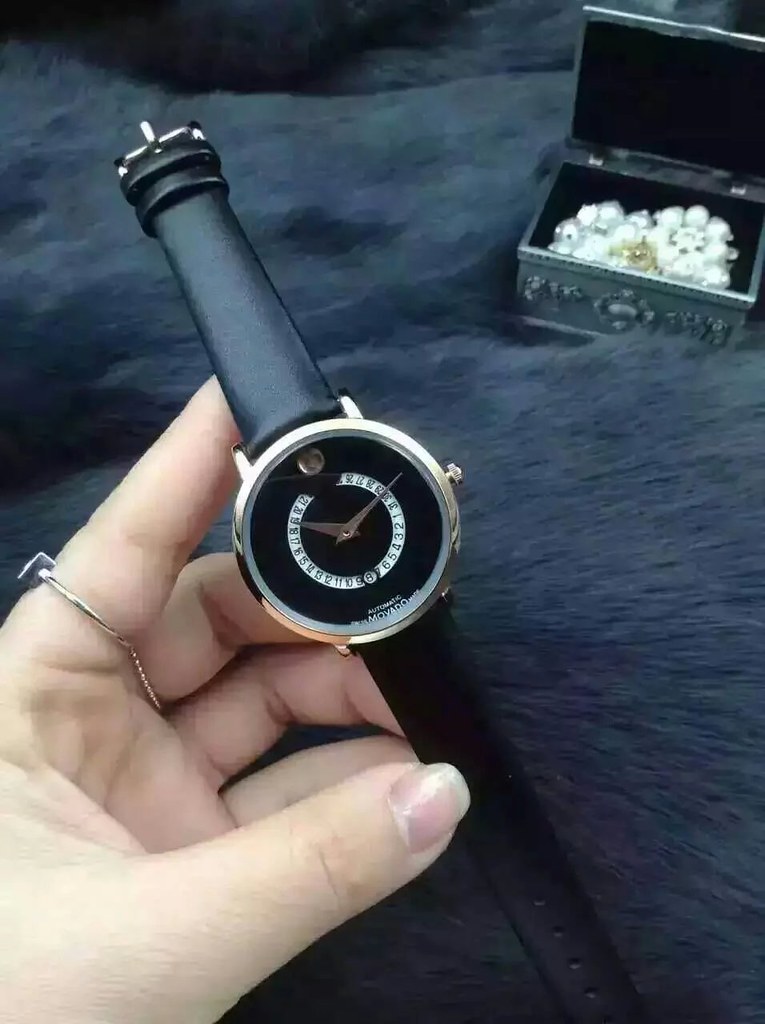The image depicts a light-skinned human hand, adorned with distinct jewelry, holding a sophisticated watch. The hand, potentially female, has a notably long thumb fingernail. It is accessorized with two rings: a silver ring on the index finger and a gold ring on the middle finger. The watch features a silver housing and a black leather band. Its face is predominantly black, distinguished by a unique design. At the top, a small, circular reflective element, possibly a stone, matches the silver tone of the housing. The watch displays time using a 24-hour format starting at 1, just past where the number 3 would typically be on a standard clock. Notably, at the bottom of the watch face, the words "Automatic Movado" are inscribed in white lettering. The background reveals a blue carpeted surface and a small jewelry box containing white beads, adding to the composition's context and richness.